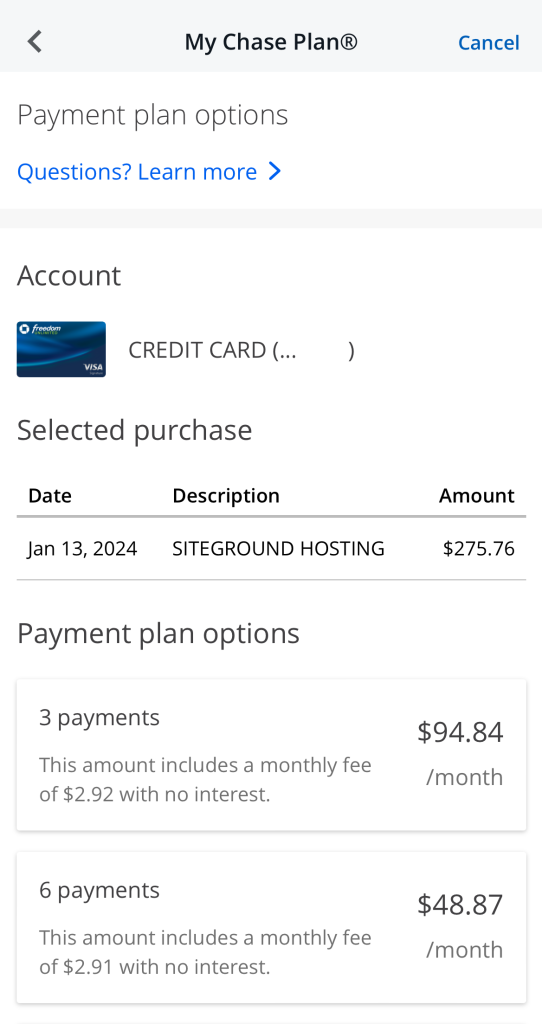**Screenshot of Chase Mobile App - Payment Plan Options Overview**

The screenshot displays the Chase mobile app interface. In the upper left corner, there is a back arrow, allowing users to navigate to the previous screen. Centralized at the top is the "My Chase Plan" trademark, and to its right is a blue "Cancel" button.

Below this top bar, there is a section labeled "Payment Plan Options." A blue hyperlink text saying "Questions? Learn More" with a right-facing arrow leads to additional information on payment plans.

The next section, marked "Account," includes a pictorial representation of a Chase Freedom credit card, accompanied by the label "Credit Card" in gray letters, followed by a redacted credit card number in parentheses.

Following this, the section labeled "Selected Purchase" details a transaction:
- **Date:** January 13th, 2024
- **Description:** SiteGround Hosting
- **Amount:** $275

Underneath the transaction details, the "Payment Plan Options" are laid out:
1. **Three Payments Plan:**
   - Includes a monthly fee of $2.92 per month with no interest.
   - Total monthly payment: $94.84.

2. **Six Payments Plan:**
   - Includes a monthly fee of $2.91 per month with no interest.
   - Total monthly payment: $48.87 for six months.

The detailed breakdown ensures clarity on how users can manage their payment plans within the app.